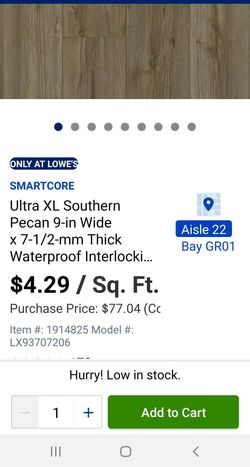Here's a detailed and cleaned-up caption for the described image:

---

This is a detailed screenshot of a product listing from Lowe's home improvement store. The upper portion of the image features a thin navy blue line running horizontally. Below this line, there's a section resembling wood flooring, showcasing a variety of light brown shades. Directly underneath the flooring section are several small circles, the first of which is navy blue, followed by eight gray circles.

On the left side of the image, there's a blue oval containing the text "Only at Lowe’s" in white. Beneath this oval, the label reads "SmartCore" in blue. Below that, it continues with "Ultra XL Sudden Pecan, Nine Inch Wide" in black, followed by "7-1/2 MM Thick, Waterproof, Interlock" and the beginning of the word “Installation,” truncated with "I...". The product is priced at $4.29 per square foot. Further down in black text, the partial phrase "Precious Price" appears, followed by a cut-off figure "$77.04,” with an incomplete parenthesis showing a “C.”

The listing further notes the item number “1914825” and model number “LX93707206.”